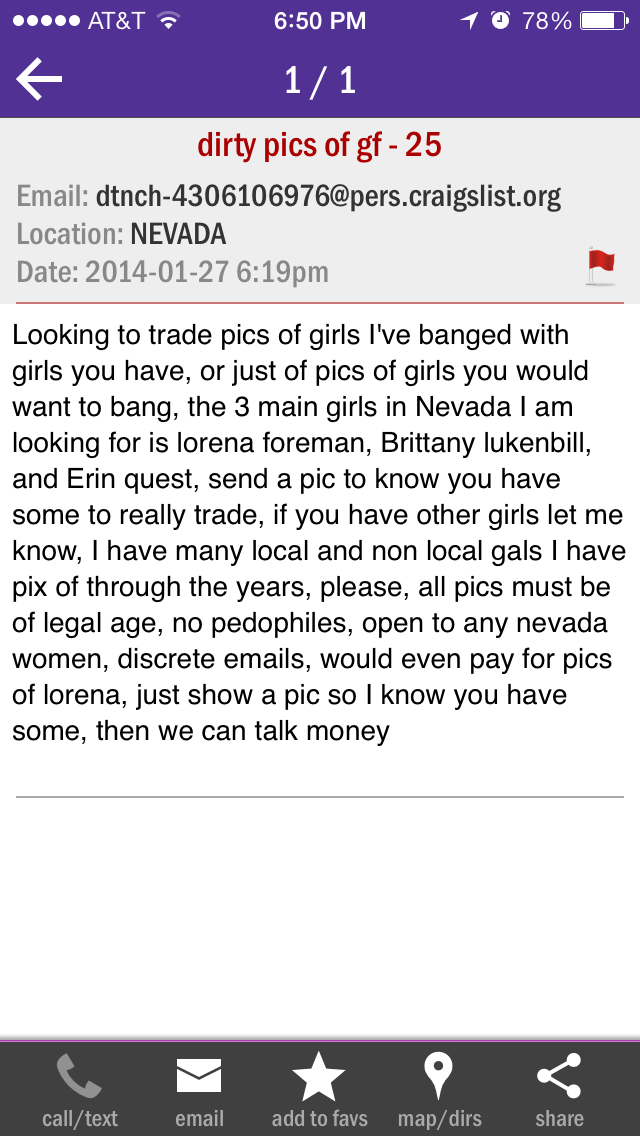The image is a detailed screenshot of a cell phone with AT&T service, displaying a purple border at the top. At the center of the top border, the time is shown as 6:50 p.m., with the battery life at 78% on the right. There's an arrow in the lower left corner of the purple border, with "1 of 1" written below it. 

The main content is an email titled "dirty pics of GF-25" in red text against a white background. The email address "dntch-4306106976@persperschragslist.org" is displayed prominently. The location is specified as Nevada in large gray letters, and the email was either sent or received on January 27, 2014, at 6:19 p.m.

The email text reads: "Looking to trade pics of girls I've banged with girls you have, or just pics of girls you would want to bang. The three main girls in Nevada I am looking for are Lorena Foreman, Brittany Lukenbill, and Erin Quest. Send a pic to know you have some to really trade. If you have other girls, let me know. I have many local and non-local gals I have pics of through the years. Please, all pics must be of legal age, no pedophiles. Open to any Nevada women. Discreet emails. Would even pay for pics of Lorena. Just show a pic so I know you have some, then we can talk money."

At the bottom of the screenshot, there's a white frame with several icons against a gray background: a phone icon, an envelope labeled "email," a star labeled "add to faves," an upside-down teardrop labeled "map/directions," and a two-pronged circle labeled "share."